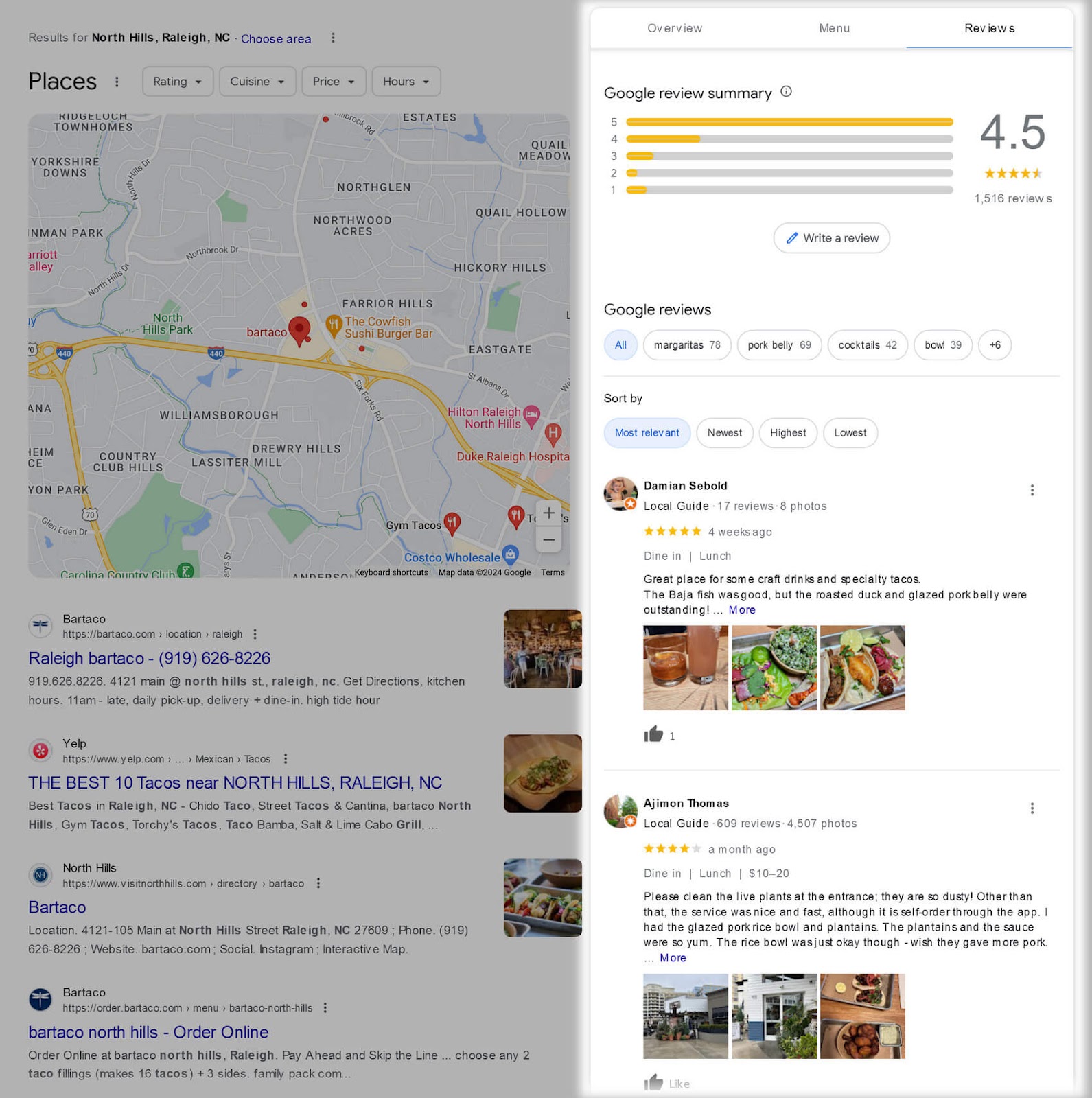In this image, we see a summary of Google Reviews for a restaurant that offers a unique dining experience with craft drinks and specialty tacos. A local guide highlighted the distinctive menu, praising the badger fish, but raving about the outstanding roasted duck and glazed pork belly. They noted an area for improvement with the dusty live plants at the entrance. The service was described as nice and fast despite being self-ordered through the app. The guide personally enjoyed a glazed pork rice bowl and plantains, mentioning that while the plantains and sauce were delicious, the rice bowl could have used more pork. Surrounding locations on the map include Northwood Acres, North Glen, Quail Hollow, Hickory Hills, Farrer Hills, Eastgate, Williamsboro, Placetown Mill, Drury Hills, Country Club Hills, and Yorkshire Downs.